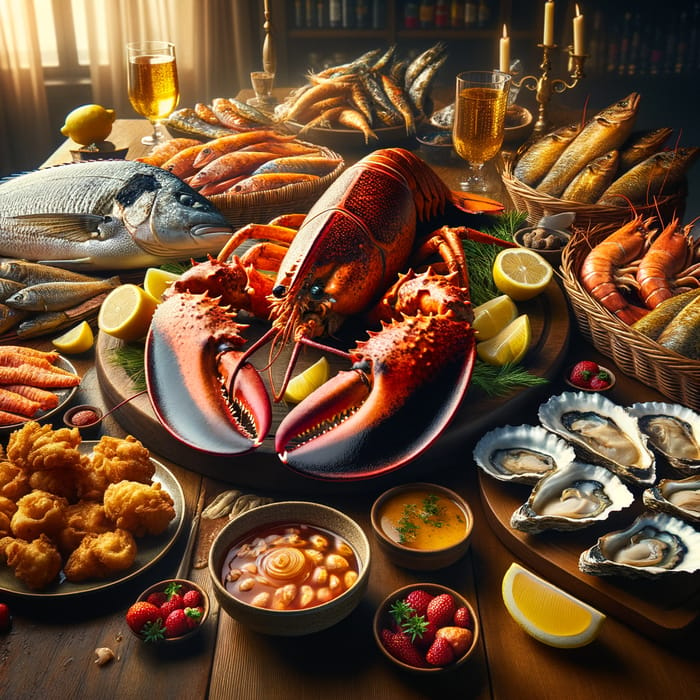This digitally rendered image depicts a lavish seafood feast arranged on a polished wooden table bathed in natural light from a nearby window. The main attraction is a large, vivid red lobster positioned on a round wooden platter at the center of the table, surrounded by sliced lemons and green garnishments. The lobster is flanked by a variety of sumptuous dishes: in the foreground are bowls of strawberries, a dip with green garnishments, a soup, and plates of fried batter items likely resembling fish and chips or fried chicken. To the right, there are platters of oysters on the half shell, mussels, and baskets containing an assortment of raw seafood including very large shrimp in hues of gray, orange, and red, and small fish. Above the lobster lies a large bluish-gray fish, while at the bottom left, you can see another platter of small, orange-hued fish. Amber-colored drinks, possibly apple cider or white wine, are scattered among the spread, casting a warm glow in the background. Overseeing the entire scene is a candelabra along with the sunlight that streams in, enhancing the intricate details of the colorful feast. A bookcase is visible at the top right, framing this abundant and inviting food display.